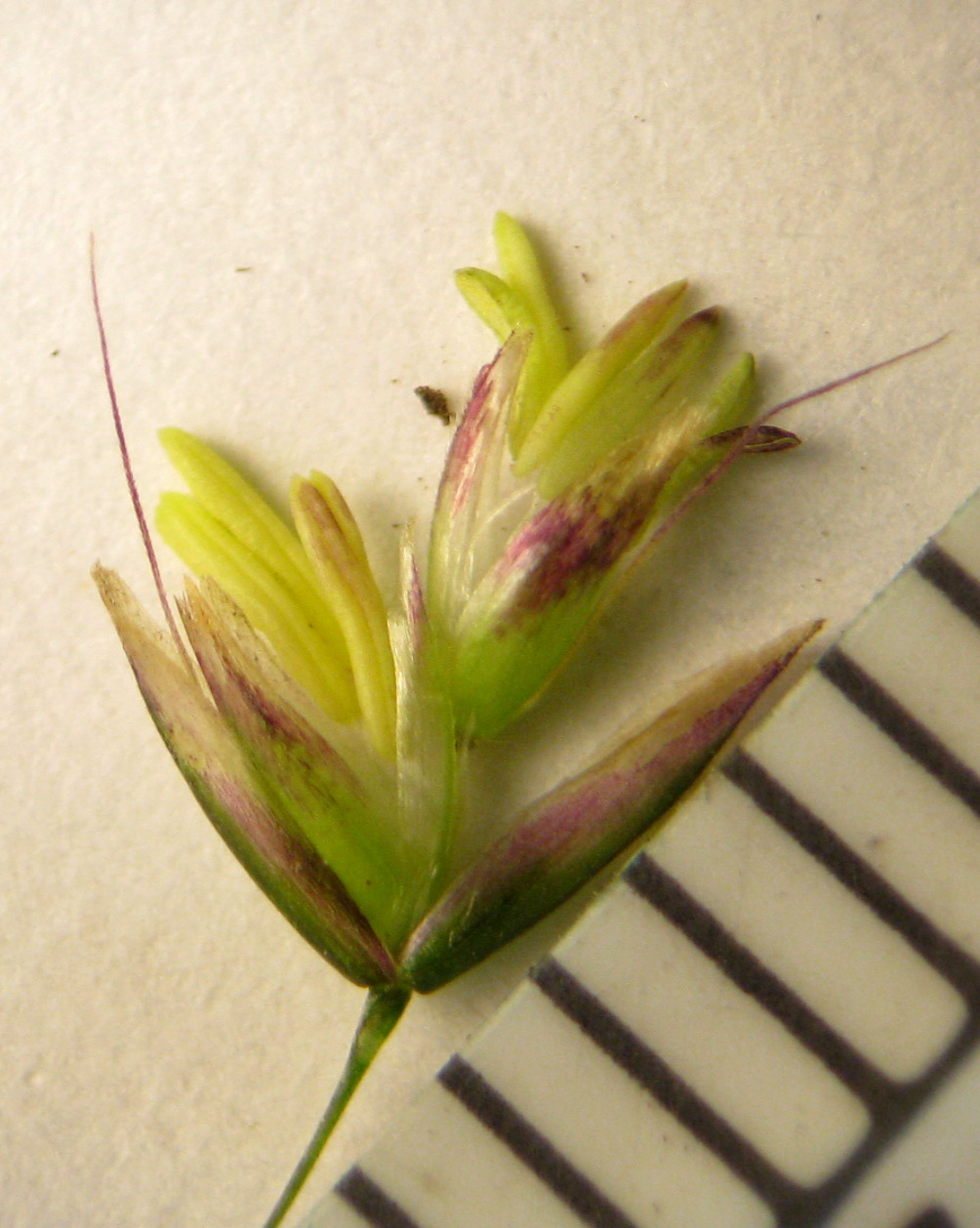The image features a close-up of a flower bud yet to bloom, set against a light cream-colored background with slight ripples. The flower's slender green stem originates from the bottom left of the frame, extending upward to the right. Midway along the stem, a cluster of leaves branches out. On the right side, there's a leaf tinged with green at the base, transitioning to purple in the middle, and accented with yellow. Adjacent to it, a couple of smaller green leaves exhibit more purple and white hues at their tips. Slightly above this cluster, three distinct yellow leaves extend to the left. 

As the stem continues, it culminates in the partially-opened bud, oriented upwards and to the right. The bud itself begins with green where it attaches to the stem, followed by purple on the right and a mix of white and purple on the left. Emerging from the bud are several thin greenish-yellow stems; three of these rise straight up but lean slightly to the right due to the flower's overall orientation. There's also a singular small purple protrusion on the right side of the bud.

In the lower right corner of the image, running parallel to the angled leaves, a ruler-like object with black lines and presumably numbers can be seen, emphasizing the scale and precision of this botanical study.